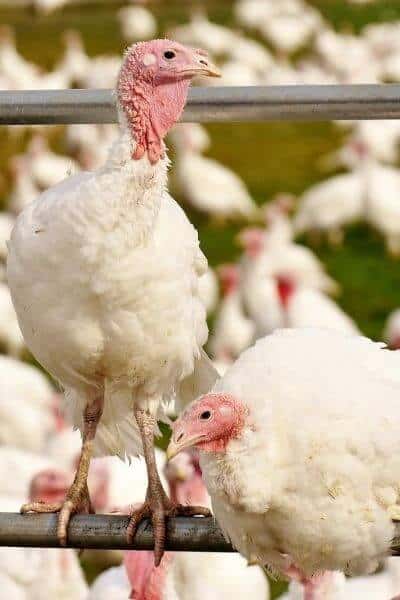This is an image of domesticated birds, likely turkeys, with two prominent ones in the foreground perched on horizontal metal bars that appear to be part of a fence. The bird on the left stands tall, displaying its light, almost white, cotton candy-like feathers, and a textured medium pink head and neck with a dark eye and a yellow-orange beak. Its long legs and claws are visible, and it looks to the right. The other bird is crouched down on a lower bar, showing similar feather and head coloration, with its head angled towards the lower left corner of the image. The background, slightly out of focus, reveals a large number of similar birds scattered across the green grass. These birds, featuring light-colored bodies and darker pink heads, enhance the impression of a densely populated bird habitat.